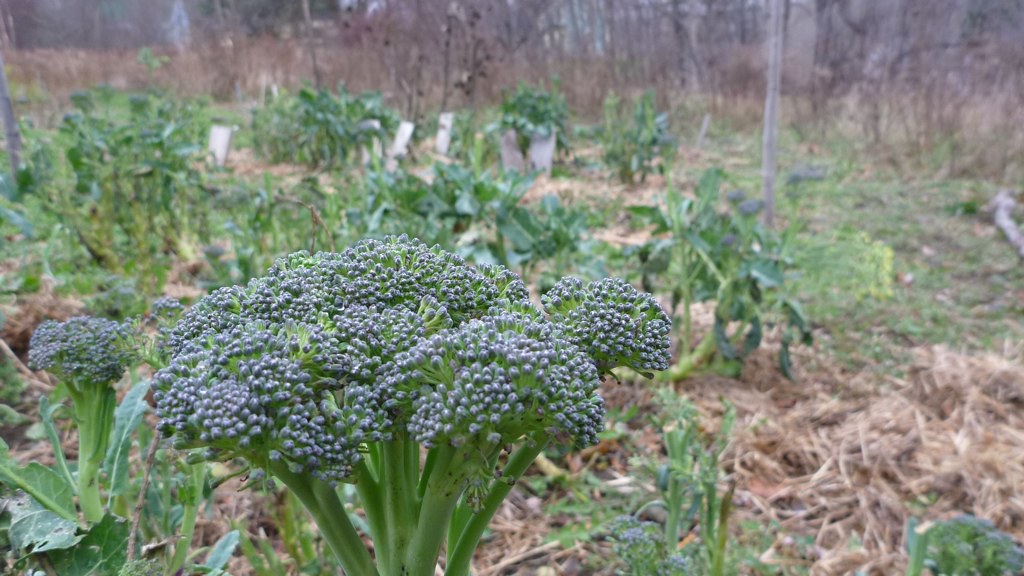This photograph captures a close-up view of a garden with a prominent head of broccoli in the lower left corner. The broccoli features a large, green stalk and a head adorned with tightly packed, bluish-purple buds. Accompanying the main broccoli are smaller broccoli plants, including one emergent head in the bottom left corner. The ground to the right is sprinkled with straw, adding a rustic touch. The background showcases a densely planted garden, mostly out of focus, where other tall, green leafy plants suggest additional broccoli or various other vegetation. Also scattered throughout are garden markers identifying different plants. In the distant background, bare trees with thin, brown branches and a white structure peeking through add depth and texture to the scene, hinting at a residential area. The image evokes the cyclical nature of gardens, preparing for a new season amidst last season’s remnants.